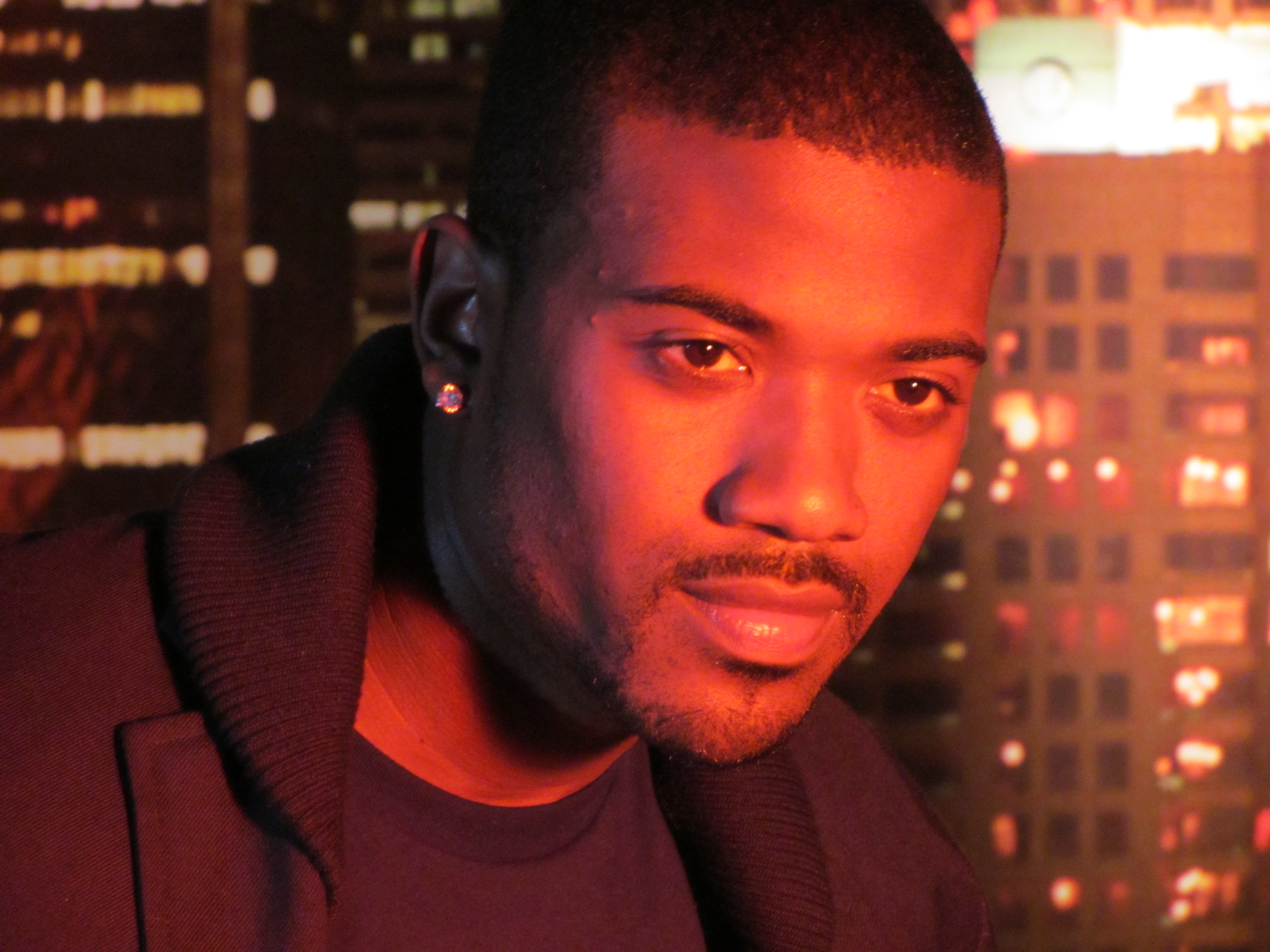The photograph captures a close-up of a man with dark skin and very short dark hair, showcasing a thin mustache and sparse facial hair, including a small goatee and a soul patch. He wears a stud earring in his visible left ear. Dressed in a dark jacket over a purple t-shirt, the man stands in front of a nighttime city skyline, seen from a high vantage point, possibly a rooftop or open window, given the absence of reflections. The scene is bathed in a red glow, likely from nearby lighting, enhancing the reflective shine on his face. Some windows in the buildings behind him are illuminated, while others remain dark. The man slightly smiles and gazes towards the right, providing a three-quarter view of his face.